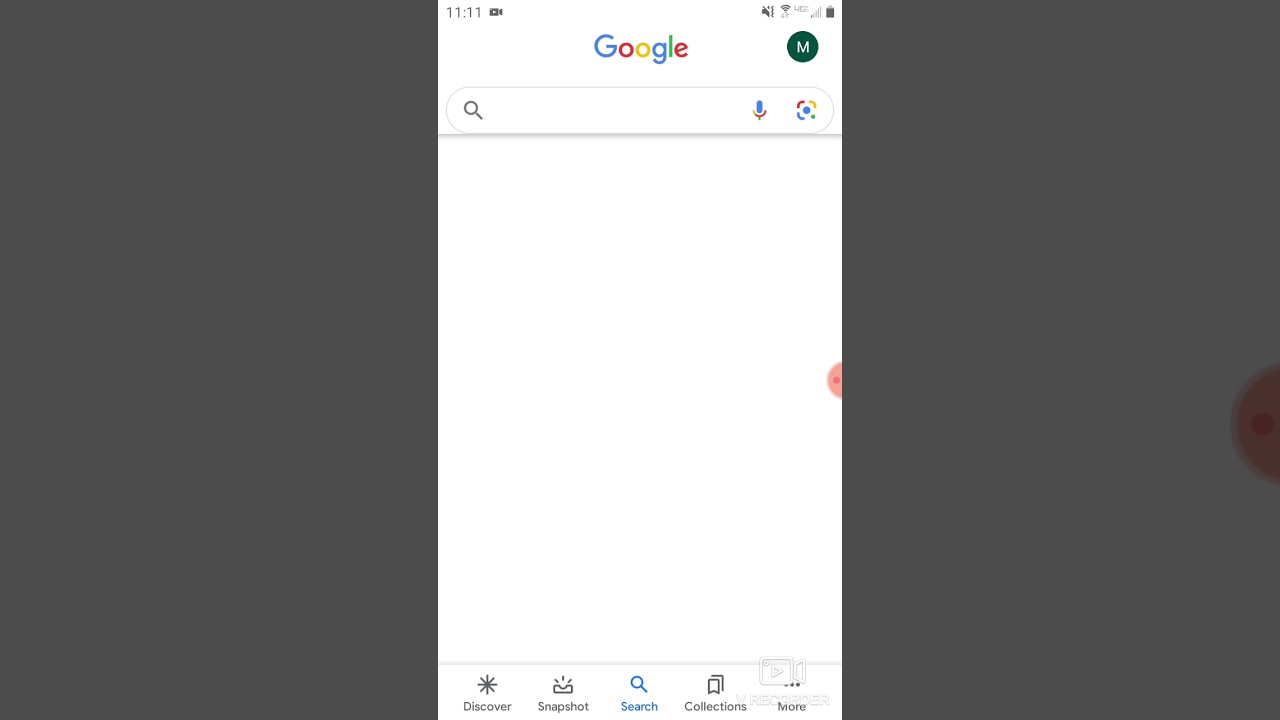This image is a screenshot of a Google search page with a minimalistic design. At the very top left corner, the time is displayed as 11:11 alongside an icon of a video camera. On the same row, situated on the far right side, there are a series of icons: a vibrate-only icon, a cell phone signal indicator, a 4G connectivity icon, a WiFi signal icon, and a battery level icon. Centrally positioned at the top is the Google logo, flanked on the far right by a green circle containing a white letter "M."

Below this header, there is a prominent search bar featuring a magnifying glass icon, a microphone icon, and a photo icon. The remainder of the page is a clean, white background, devoid of any additional content.

At the bottom of the screenshot is a navigation bar with options labeled from left to right as Discover, Snapshot, Search, Collections, and More. Notably, a translucent pink circle hovers near the right edge, positioned at the center-right of the screen.